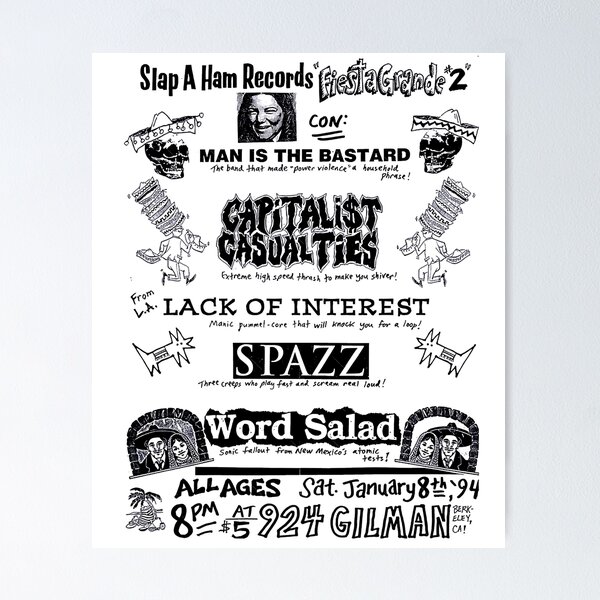Here is a detailed and cleaned-up caption for the image:

---

A black and white poster advertising the Slap a Ham Records Fiesta Grande 2 event held on Saturday, January 8th, 1994. The design is monochromatic, with various detailed illustrations and text. The poster's headline reads, "Slap a Ham Records Fiesta Grande 2," and prominently features an image of a man. Beneath the headline, it lists the performing bands with the prefix "con:" Man Is the Bastard, Capitalist Casualties, Lack of Interest, Spaz, and Word Salad.

The event is marked as open to all ages and took place on Saturday, January 8th, 1994, at 8 p.m. at the iconic venue 924 Gilman in Berkeley, California, with an entry fee of $5.

The poster includes various intricate images: a skull adorned with a sombrero, a man walking away while wearing multiple sombrero hats, and a stylized dog seemingly constructed from stars. Additionally, at the bottom near the name "Word Salad," there is an illustration of a man and woman, and another depicting a traditional Mexican family consisting of a husband and wife.

---

This caption reflects the descriptive and organized nature of the poster, providing a clear and detailed summary of its content.